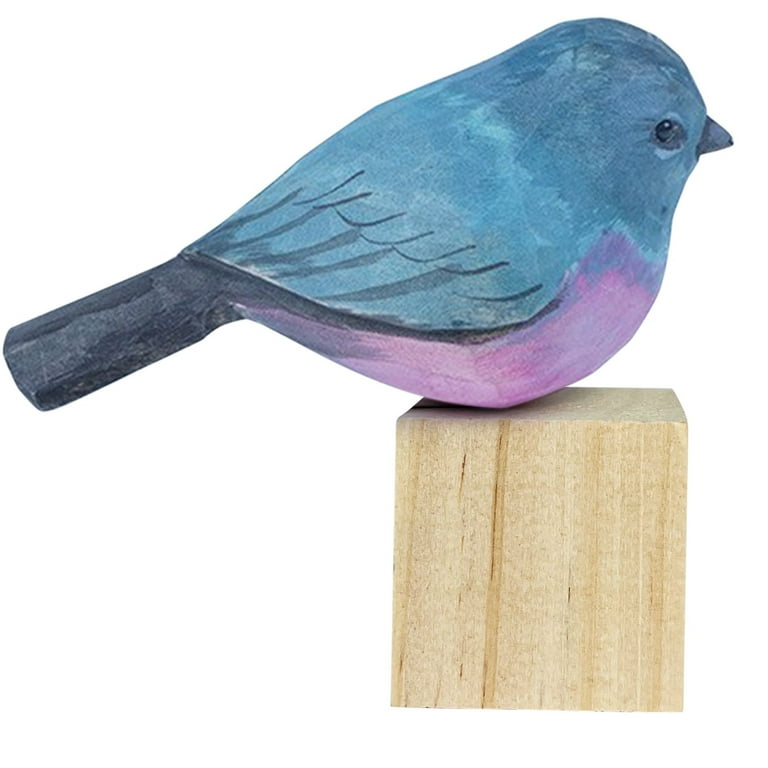This image portrays a handcrafted wooden bird figurine, perched on an unadorned wooden block serving as its stand. The bird, modest in size, exhibits a simple yet detailed design with intentional brush strokes visible on its surface. Its primary color is a vivid blue, transitioning to a hint of pink on the lower body, while the beak and tail are painted a dark purple or black. The bird’s wings are delineated with black lines, and it features a small eye. With a blunt, rounded tail, the figurine lacks feet and lies flat on its stomach atop the square wooden base. The background of the image is completely white, providing no sense of scale or context, but the bird could resemble a small species such as a sparrow or a common finch.